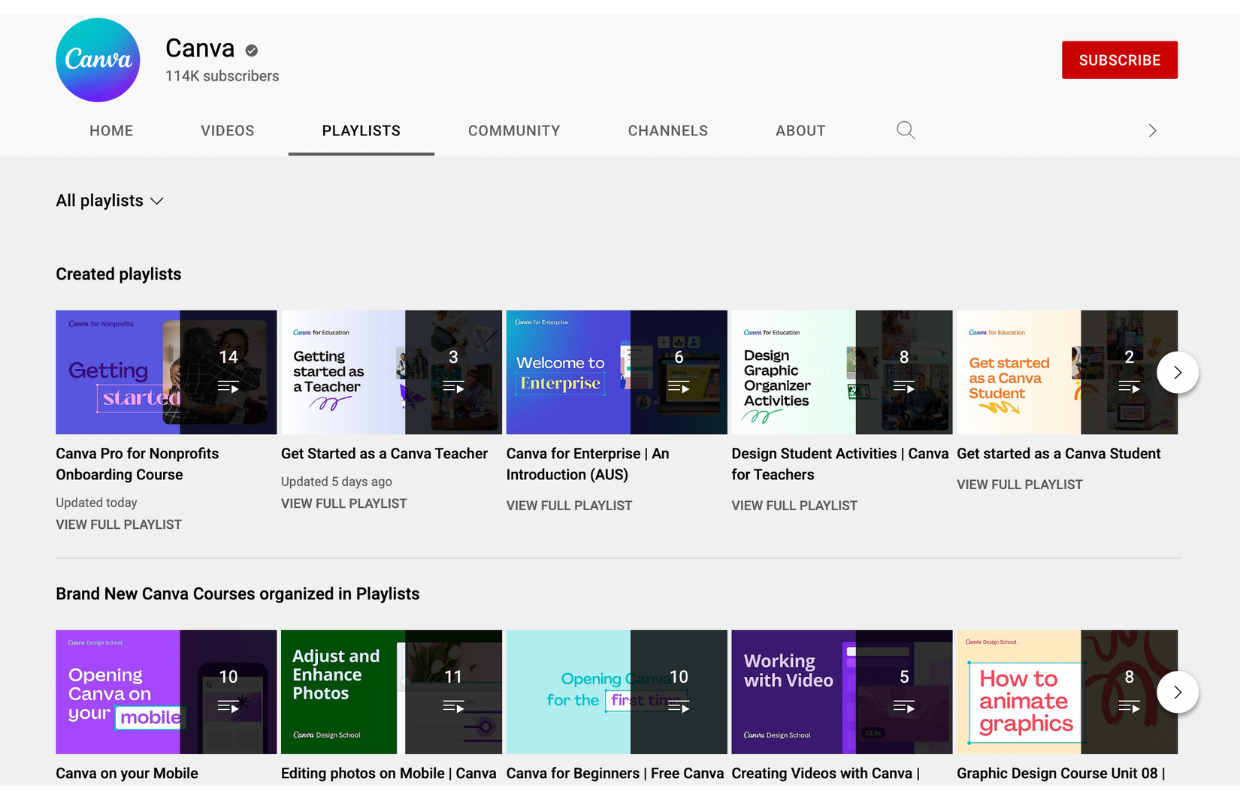The image depicts the homepage of the Canva YouTube channel. At the top left, the Canva logo is displayed within a turquoise and blue circle. To the right is the channel name "Canva" with "114k subscribers" displayed underneath. On the top right corner, there is a red rectangular "Subscribe" button. The top background is light gray. 

The navigation menu, located below the header, features six categories from left to right: "Home," "Videos," "Playlists," "Community," "Channels," and "About." Below this menu, the phrases "All Playlists" and "Created Playlists" are highlighted. Five created playlists are displayed, with their respective video counts: the first playlist has 14 videos, the second 3 videos, the third 6 videos, the fourth 8 videos, and the fifth 2 videos.

The playlist titles are as follows:

1. Canva Bro for Nonprofits Onboarding Course
2. Get Started as a Canva Teacher
3. Canva for Enterprises and Introduction
4. Design Student Activities: Canva for Teachers
5. Get Started as a Canva Student

Beneath these playlists is a section titled "Brand New Canva Courses Organized in Playlists," again listing five playlists with their respective video counts: 10, 11, 10, 5, and 8 videos from left to right. The entire layout is set against a light gray background. Notably, on the right edge of the last playlist, there is a white circle with a mini arrow inside it, centrally positioned.